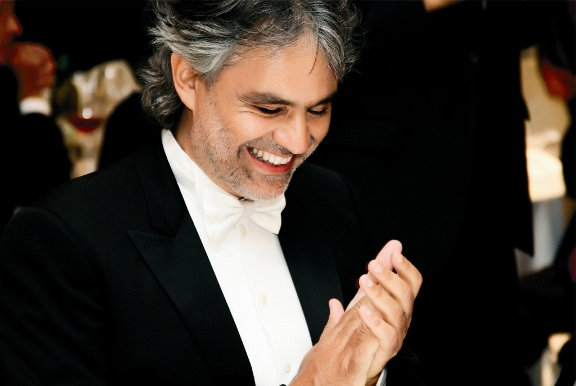In this indoor photograph, which is about four inches wide and three inches tall, we see an older gentleman of lighter, possibly light brown, skin, and perhaps of Italian descent, dressed in a formal black tuxedo with a white shirt and white bow tie. The image captures him from mid-chest up to just below the top of his head, which extends off-screen. His graying, slightly disheveled hair and salt-and-pepper stubble hint at a casual elegance. His downcast eyes, possibly closed, show him looking down as he smiles broadly, his white teeth visible. His hands are clasped together as if he has been clapping, with his left palm inside his right hand. Behind him, the dimly-lit background suggests a formal event, such as a black-tie or white-tie affair, with glasses of wine and others in similar attire. Notably, a figure in the upper left corner appears similarly dressed, standing beside a table with a white tablecloth, adding context to the celebratory environment. The overall color scheme of the photograph is dominated by blacks, whites, and grays, giving it a sophisticated and classic feel.